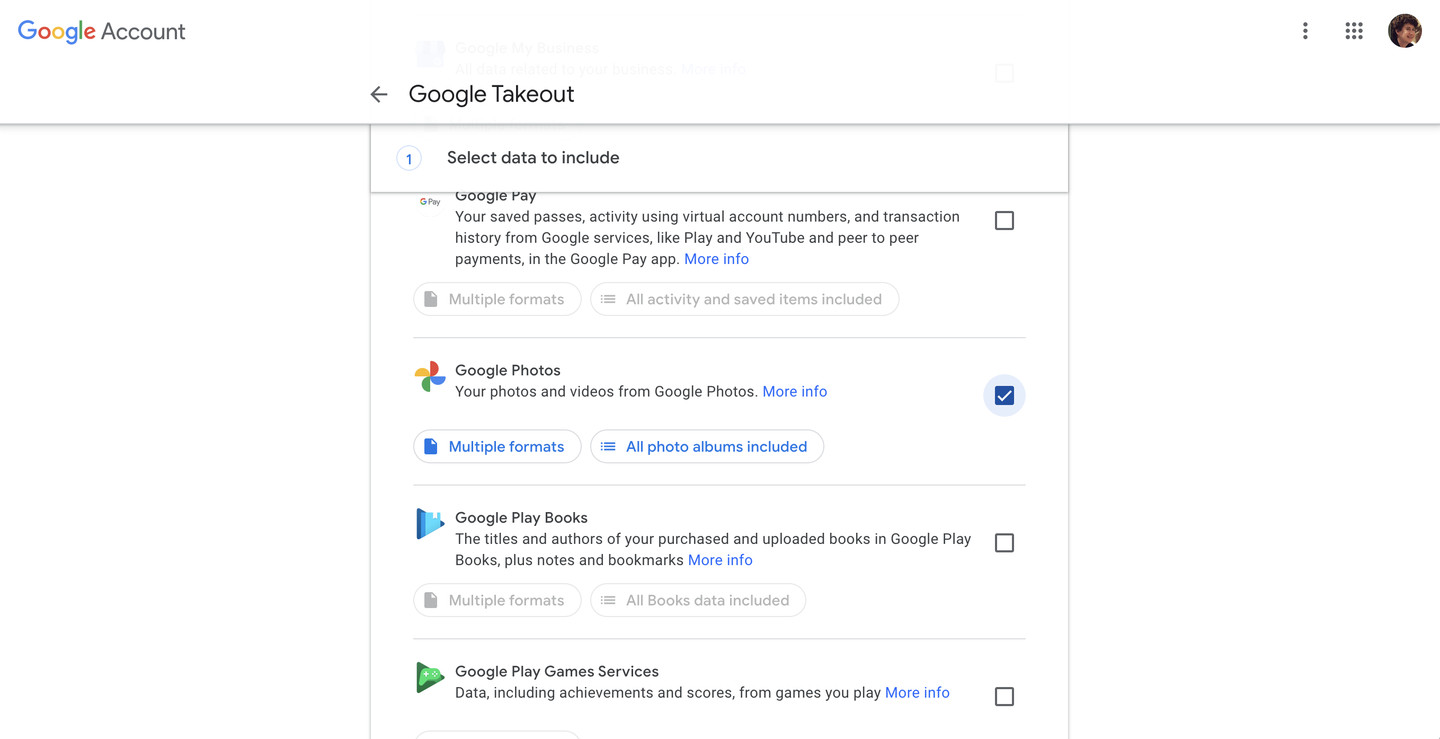This screenshot captures the interface of Google Takeout, a service that enables users to download data from their Google Account. The topmost section features a header with essential navigational elements: a 'Google Account' label, a back arrow icon adjacent to the 'Google Takeout' title, a user profile picture on the right, along with the Google Apps grid icon and a vertical ellipsis (three vertical dots) for additional options. Below this header, the section titled 'Select Data to Include' is prominently displayed.

The main content area lists various data types, including Google Pay, Google Photos, Google Play Books, and Google Play Game Services. Notably, only the checkbox next to Google Photos is selected. The interface boasts a clean and user-friendly design, characterized by a white background and black text, emblematic of Google's consistent design philosophy across its products. 

Interactive elements are highlighted by blue text and icons, guiding the user experience. Checkboxes beside each data type allow users to choose specific datasets for download. Additional information about each data type is accessible via 'More info' links. Once the selection is made, users can download the chosen information, which will be sent to their email. This ensures a streamlined process for exporting personal data from the Google ecosystem.